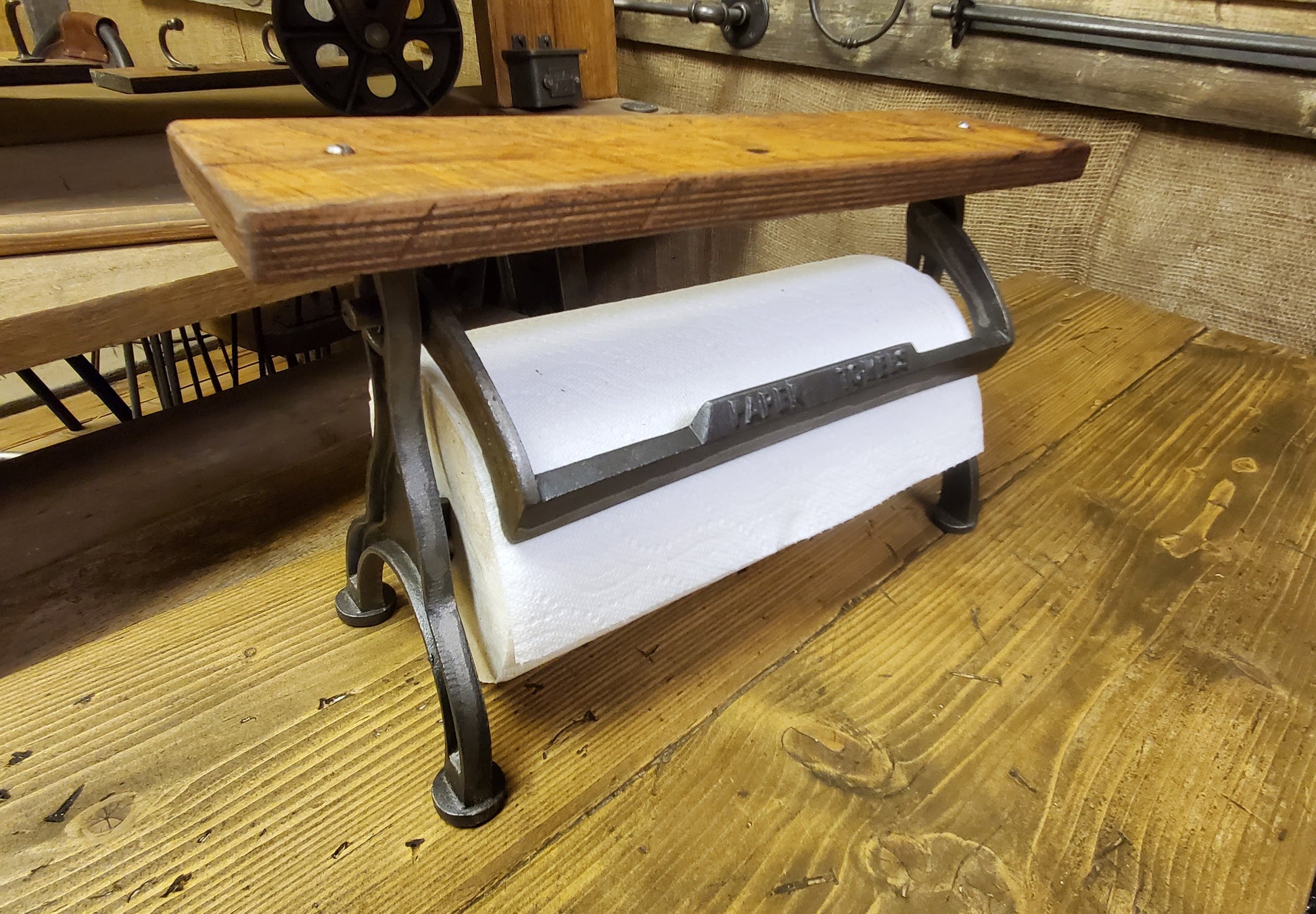This photograph depicts an antique-style paper towel holder positioned centrally on a wooden countertop. The holder features a top section made of brown wood and a bottom section composed of black iron, crafted to securely hold the white paper towels. Two silver bolts are visible, securing the wooden structure. Surrounding the image are wooden floorboards and walls, contributing to the rustic ambiance. The upper left corner of the image showcases a circular metal item that resembles a spool for clothesline wire, complete with holes around its border. Additional metal hooks and hanging fixtures are present in the background, hinting at more cast iron items designed for organization. The intricate wood grain pattern and the classic, aged design of both the paper towel holder and the surrounding furnishings suggest a setting reminiscent of an old-fashioned store or workshop.